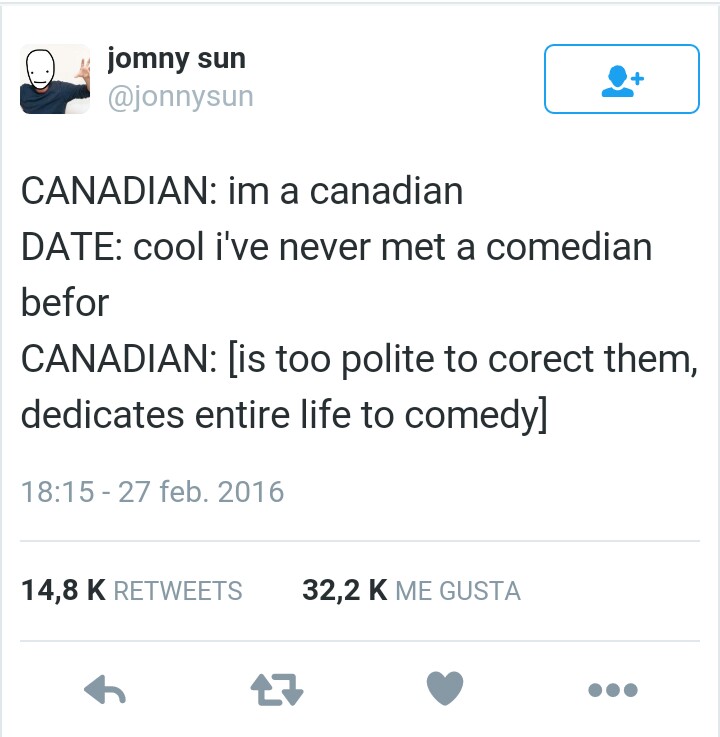Here’s a cleaner, detailed caption for the described image:

---

**Screenshot of a Simplified Twitter Post**

At the top of the screenshot, a tweet from a user named John is shown. The username reads "JohnJohnMeetJohnny," but "Johnny" is uniquely spelled as "J-o-m-n-m-n-y." Below this, the handle is displayed as "@Johnnys_son," with "Johnny" correctly spelled with two 'n's.

The image embedded in the tweet features a simplified drawing of a human figure. The figure has an ordinary body with arms raised in the air and a very basic facial illustration, characterized by dot eyes.

The tweet text reads in all lowercase: "canadian" followed by a line, "im a canadian." Below that, it continues: "cool, ive never met a comedian before," with the word "before" missing the final 'e'. Another line states: "canadian [is] too polite to correct them, dedicates entire life to comedy."

The timestamp of the tweet is "18:15, 27th of February," followed by a seemingly erroneous year "14,000." The post has garnered significant interaction, boasting 800 retweets.

---